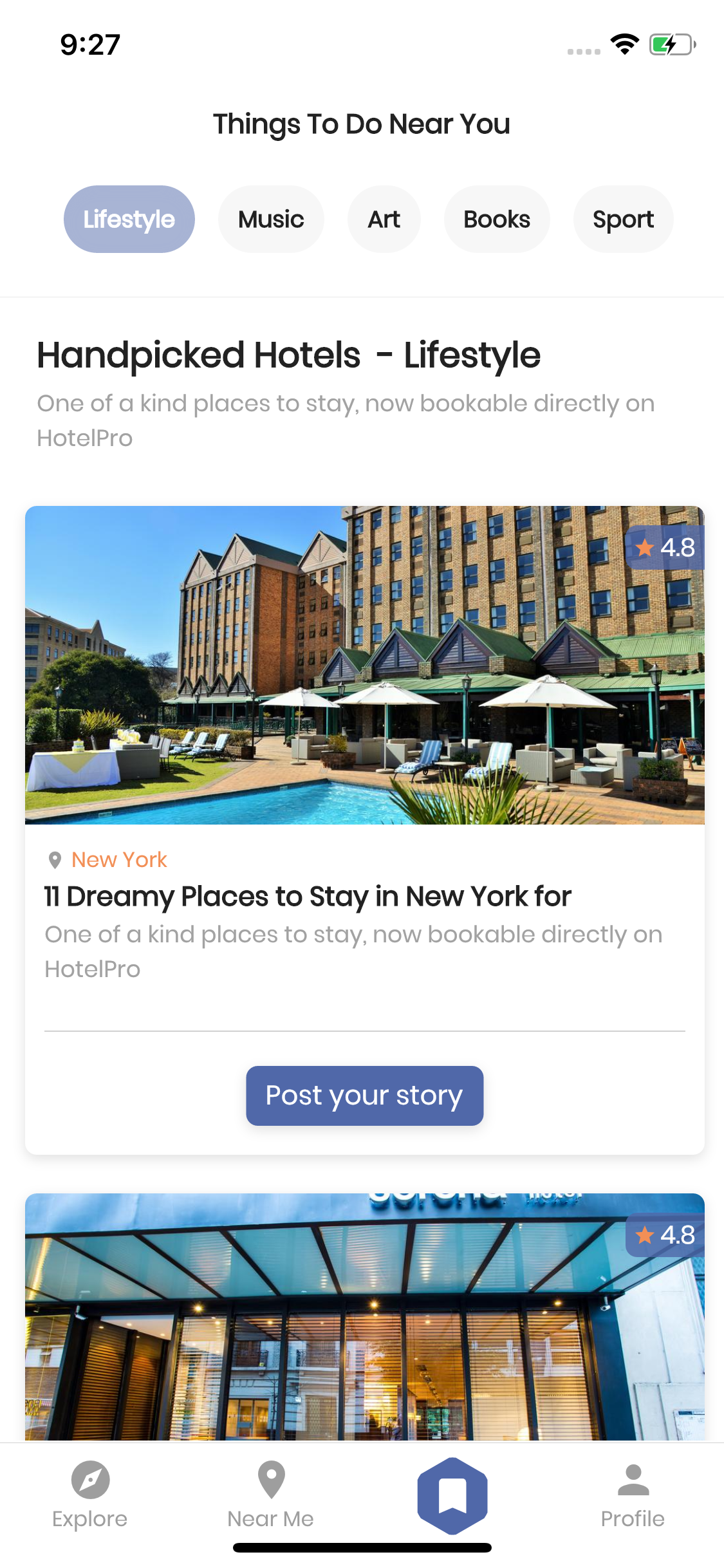This is a screenshot taken from a mobile phone displaying an app interface. The background is white. In the top left corner, the time is shown as 9:27, accompanied by a battery icon that is approximately halfway full. Below this, a section titled "Things to do near you" is visible, featuring various clickable tabs. The currently selected tab is "Lifestyle," highlighted in light purple, while the other tabs—"Music," "Art," "Books," and "Sport"—are gray.

The following section, labeled as "Hand-picked hotels - Lifestyle," features a promotional blurb: "One-of-a-kind places to stay now bookable directly on Hotel Pro." This is accompanied by an image of an upscale hotel, showcasing a pristine pool area with chairs and umbrellas against a backdrop of a clear blue sky.

Further down, there's a heading: "New York: 11 dreamy places to stay in New York for a one-of-a-kind experience." This caption is mirrored below the hotel image, reiterating the availability of unique accommodations bookable through Hotel Pro.

At the bottom, there's a prominently featured blue button labeled "Post your story," and nearby, a smaller image of some windows.